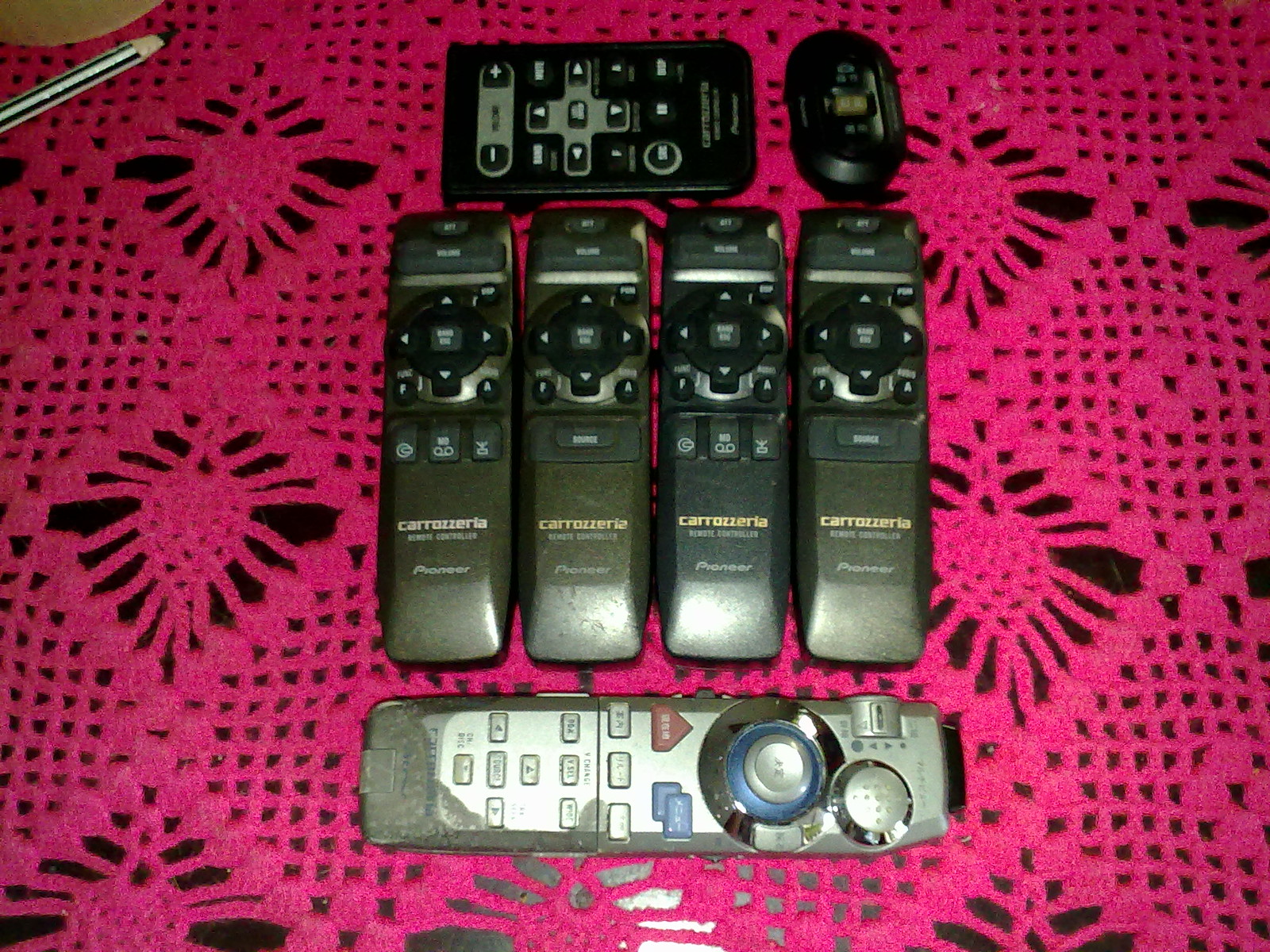This vibrant photograph, taken from a bird's-eye view, captures a textured scene on a tabletop. A striking neon pink, knitted lace tablecloth with intricate patterns and both large and small holes covers a dark brown table surface, peeking through the threads. In the top left corner of the image rests a silver pencil with a black tip. Centrally placed on the tablecloth are seven remote controls organized meticulously. There are four vertically aligned, identical TV remotes branded with 'Carozzeria' in the middle. Below these, a slightly worn silver TV remote is positioned horizontally. Above them sits a smaller, possibly more beat-up remote for a different device, also horizontally placed. The overall arrangement highlights the varied appearances and conditions of these remotes, all set against the vivid backdrop of the lace tablecloth.